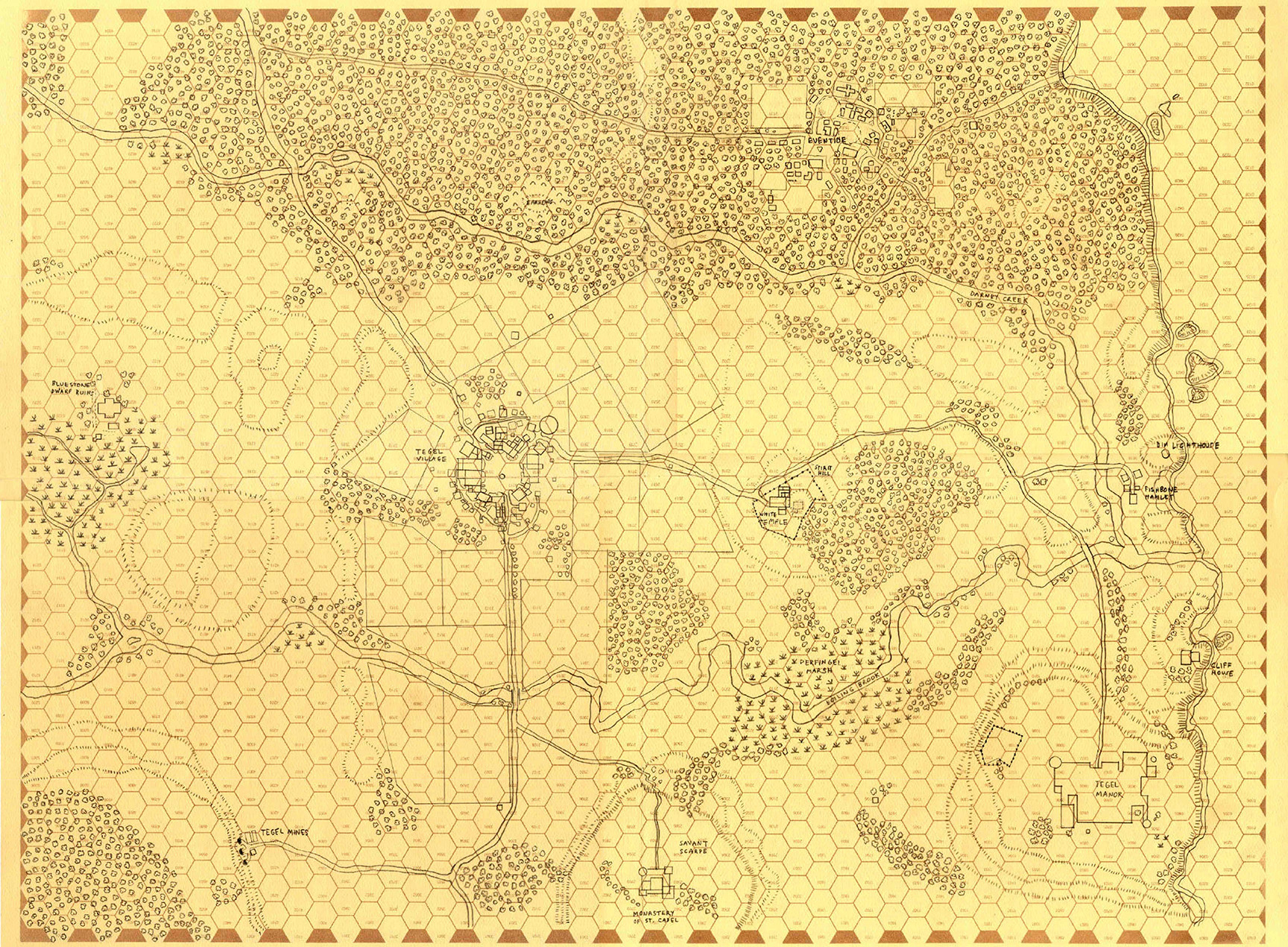The image features an intricate map-like illustration set against a dull yellow background, characterized by a repetitive honeycomb pattern. The map, which might depict a piece of land or a gaming board, is divided into numerous hexagonal cells. Scattered across the map are densely packed areas of trees, streets, and multiple small buildings, with one notable isolated building situated in the lower right corner, interconnected by a network of roads. Surrounding the primary map is a decorative border composed of brown parallelograms and triangles, adding to the image's ancient or traditional aesthetic. The map includes various squares, circles, and possibly letters or numbers, though the text is too small to discern clearly.